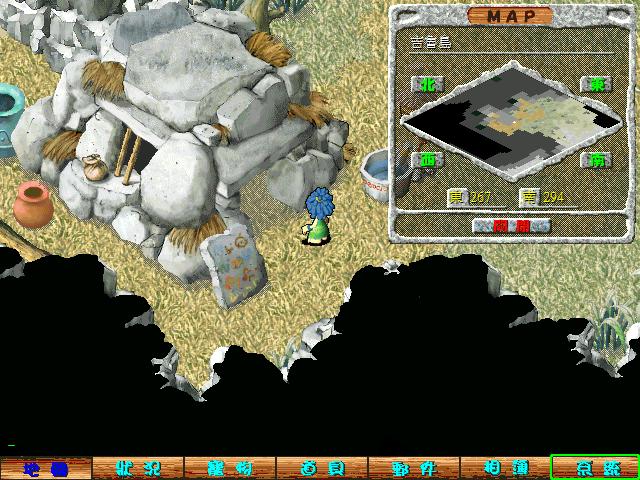The screenshot captures a scene from a computer game. The main focus is a cave-like stone house built from piled rocks, with straw visible in the gaps between them. The house has window-like openings with sticks resembling bars. Adjacent to the house, multiple clay pots and vessels are scattered around, along with a stone marker adorned with hieroglyphics or possibly similar markings. A character with blue hair, clad in a green outfit, stands outside the stone structure on a sandy terrain. In the upper right corner of the image, a map is displayed, featuring numbers and Japanese characters. The bottom section of the image displays additional elements with brown and black backgrounds, and more Japanese characters. The surroundings give an impression of a coastal setting, contributing to the game's immersive environment.